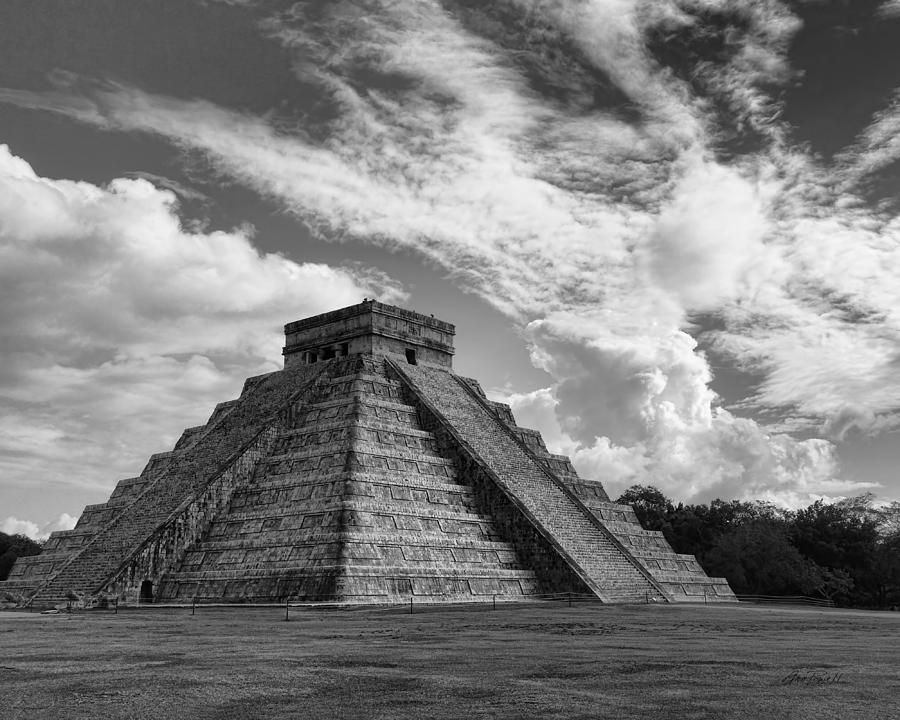This black and white photograph captures a majestic ancient pyramid, likely of Mayan or Aztec origin, with distinct boxy, prism-shaped architecture and a flat-roofed structure at the summit. Taken from a low vantage point, the image emphasizes the monument's grandiosity and height, showcasing its nine tiers and the central staircase that ascends to the top on each visible side. The scene is set on flat terrain that appears to be either grass or dirt, enclosed by a simple rope fence. In the background, clusters of trees and bushes encircle the area, extending to a distant tree line. The sky above is filled with fluffy, wispy clouds, providing a striking contrast against the dark sky, which spans the upper portion of the image. This powerful depiction highlights both the intricate details and the impressive scale of the ancient structure.